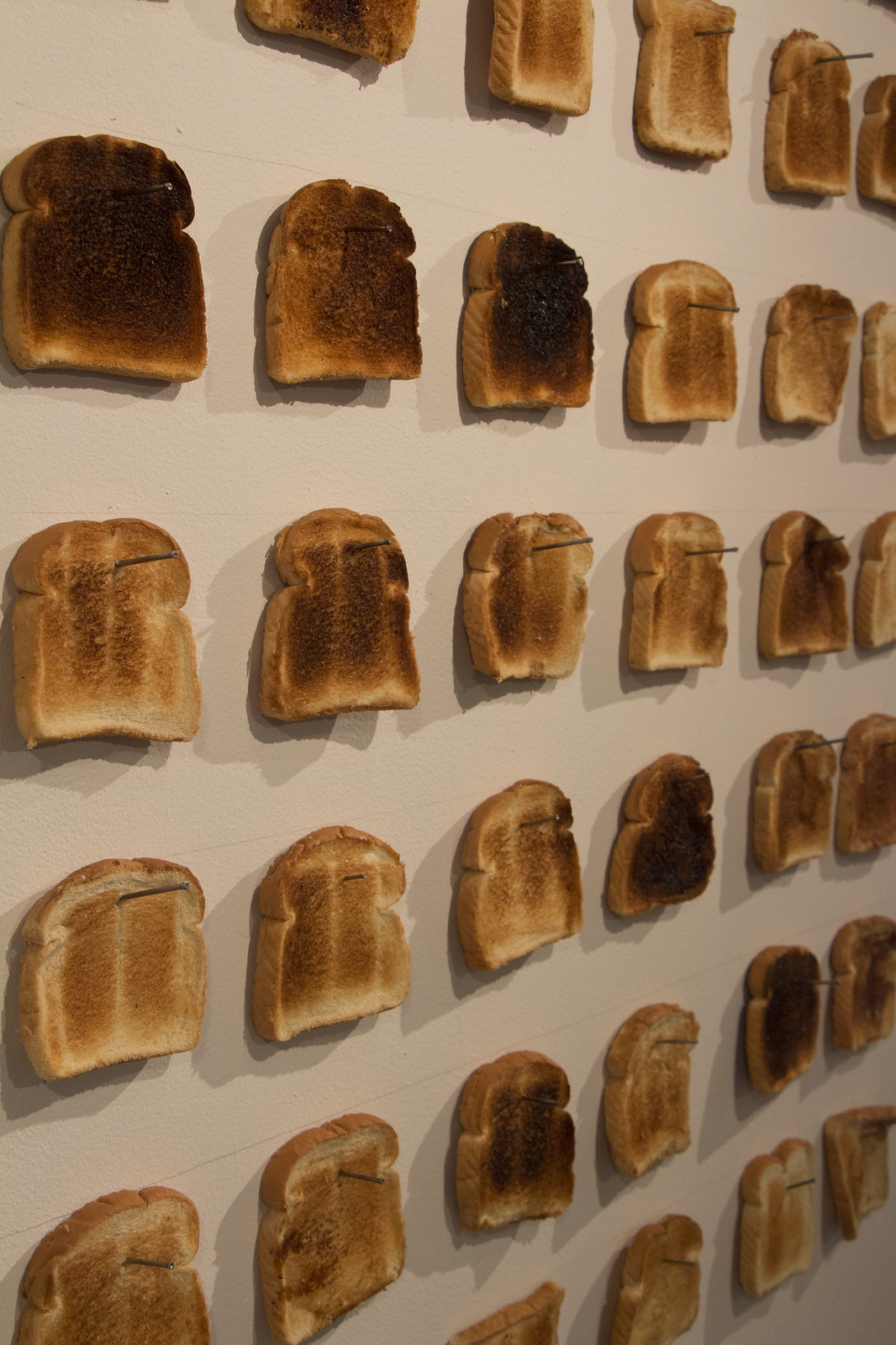This photograph portrays a meticulously arranged art installation of approximately 30 pieces of toast, evenly spaced and nailed to an off-white wall. The toast slices are organized into six neat rows and columns, with each slice secured by a long nail. The toast displays a spectrum of doneness: some slices are light tan, others are a medium brown, while several are almost entirely blackened. The lighting suggests an indoor setting, and the various degrees of toasting create distinct patterns of shading on the wall. The image captures the texture and contrast of the bread, highlighting the diversity in toasting levels from slightly toasted to charred black.